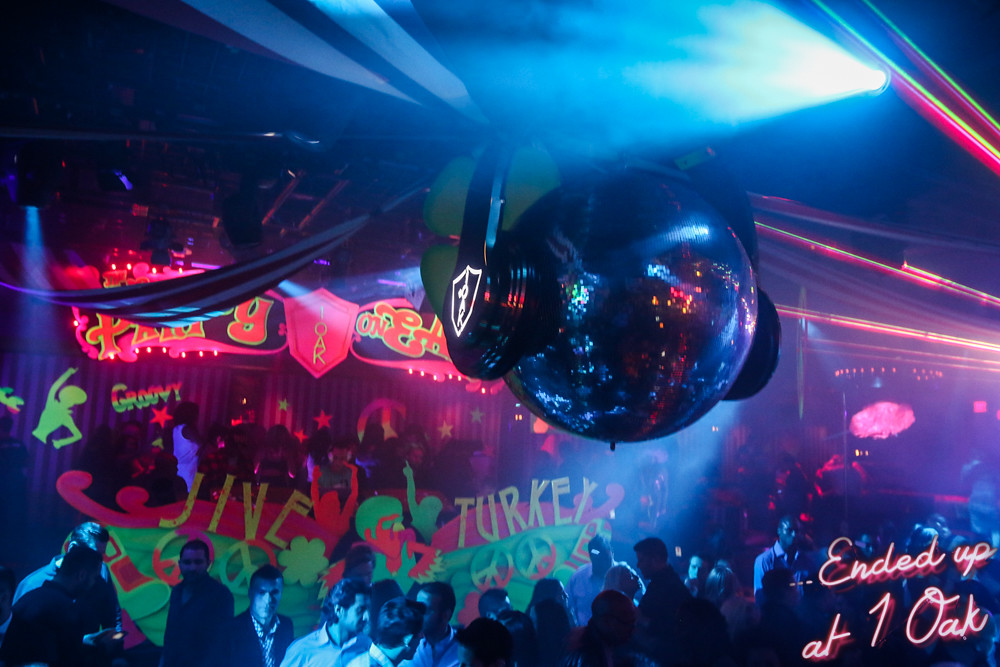This vibrant nightclub photograph captures a lively scene from above, showcasing a dynamic mix of details glowing under colorful lights. Dominating the center, a large disco ball adorned with over-ear headphones reflects hues of pink, green, and blue. The ceiling and various lights form a luminous canopy overhead. Below, partially visible people fill the frame, mingling in front of vividly illuminated decorations. Prominently displayed are neon-colored peace signs, stars, and the phrase "Jive Turkey" in bright letters. Adding to the retro atmosphere, the word "Groovy" is visible among the decorations. In the bottom right corner of the image, a striking neon-style text reads "Ended Up at One Oak," enhancing the playful, nostalgic vibe of this immersive club scene.